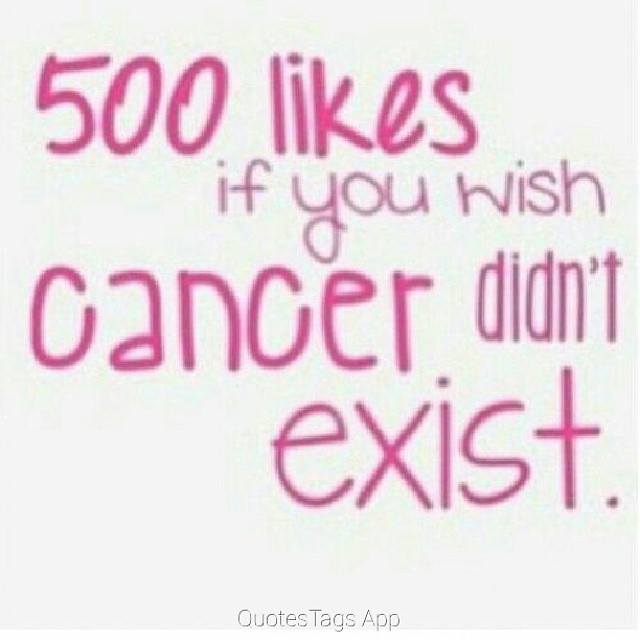The image depicts a simplistic digital graphic likely crafted through an app, featuring a white square background with pixelated and blurry text in varying shades of pink. The central message reads "500 likes if you wish cancer didn't exist," where the words "500 likes" and "cancer" are particularly bold and thicker compared to the rest. The font is a bubbly, girly, and somewhat swirly style, exclusively in lowercase letters with inconsistent sizing and thickness, giving it a hand-drawn appearance as if manipulated by a computer program. At the bottom of the image, there is a subtle watermark-like text that reads "quotes tags app," suggesting the tool or platform used to create the graphic. This type of post appears tailored for social media, designed to garner likes and shares for awareness. The image contains no other visuals, focusing entirely on the impactful text against a stark white backdrop.